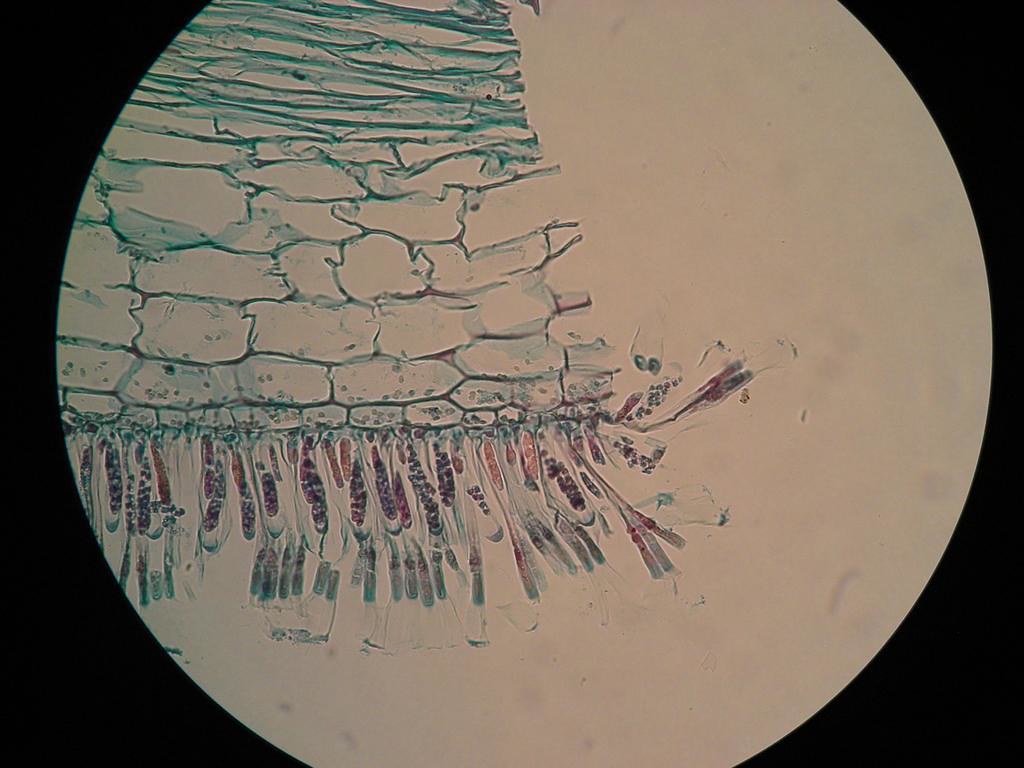The artwork in this rectangular image features a striking full moon, centrally placed against a solid black background. The moon appears meticulously painted, predominantly white, with intricate designs suggesting a mix of turquoise stone walls and mysterious flora. In the left section of the moon, these turquoise stone walls are depicted with stones stacking progressively smaller towards the top. Complementing this, small purple flowers and intertwined ballet slipper-like ribbons cascade from the base of the wall. Near the right-center, a pair of sunglasses discreetly emerges, blending into the ethereal lunar surface. The piece employs a palette of black, white, blue, and purple, and its fluid, somewhat abstract execution hints at watercolor techniques. The overall composition evokes the intricate world of a telescope or perhaps the magnified view under a microscope, capturing an unusual, otherworldly scene.